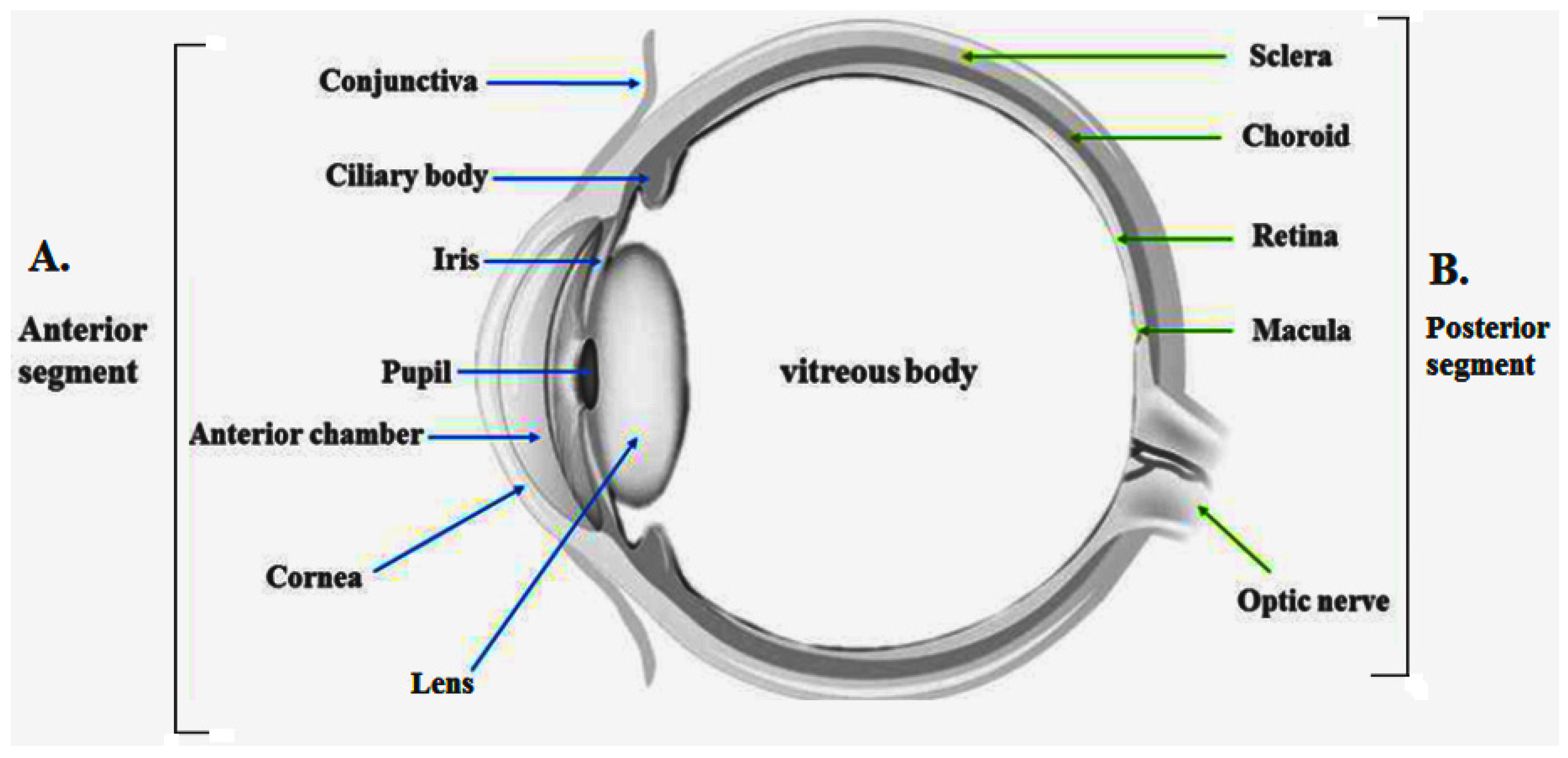This detailed infographic depicts a side view diagram of an eyeball, meticulously labeling its anatomical components. The image is predominantly in gray and white, with black text prominently highlighting the vitreous body at the center. The diagram is organized into two main sections: the anterior segment and the posterior segment. 

The anterior segment, marked with blue arrows, includes the conjunctiva, ciliary body, iris, pupil, anterior chamber, cornea, and lens. Conversely, the posterior segment, indicated by green arrows, outlines the sclera, choroid, retina, macula, and optic nerve. Each of these components is clearly labeled, providing a comprehensive overview of the eye's structure.